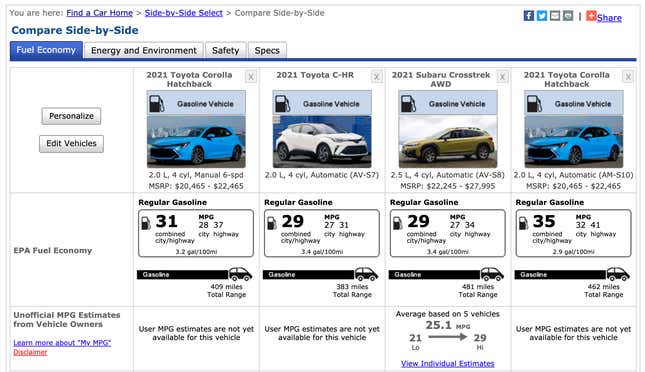In this screenshot, the image showcases a website dedicated to car information against a solid white background. In the upper left corner, there is a "Find a Car Home" link, indicating the primary navigation point. Adjacent to it, the option "Compare Side by Side" is selected and underlined in blue, suggesting its active status. Below this navigation bar, several tabs are visible, including "Fuel Economy," "Energy and Environment," "Safety," and "Specs," organized for easy access to different categories of information.

In the upper right corner of the page, icons for social media sharing (Facebook and Twitter), email (represented by a white envelope), and a general share button are present for convenience. 

The main content area highlights a comparative section, beginning with the "Fuel Economy" tab, which is dark blue, suggesting it’s the active tab. The subsequent tabs are "Energy and Environment," "Safety," and "Specs," arranged in sequence.

The page features four colored photographs of different cars, each labeled with their respective models. These include the 2021 Toyota Corolla Hatchback, the 2021 Toyota C-HR, the 2021 Subaru Crosstrek AWD, and again the 2021 Toyota Corolla Hatchback, specifically noted as a gasoline-powered vehicle.